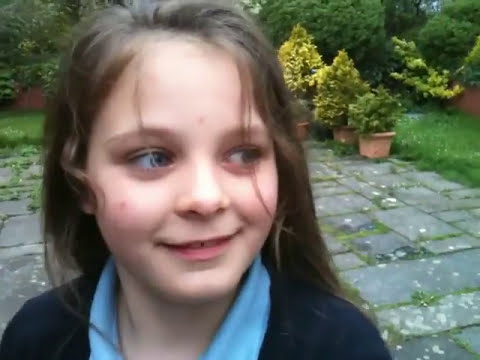This daytime outdoor photograph captures a young girl, approximately 8 or 9 years old, with shoulder-length brown hair and pale skin. She is smiling and looking slightly off to the right, giving her a happy or quirky expression. The girl wears a light blue shirt underneath a darker, almost black shirt. Behind her, gray flagstones, slightly overgrown with grass, are arranged on a lush green lawn. Three terracotta clay vases with small bushes are placed on the flagstones, adding texture and color to the scene. In the farther background, the photo showcases the vibrant greenery of a lawn, a tree, and more foliage, evocative of a serene garden setting.